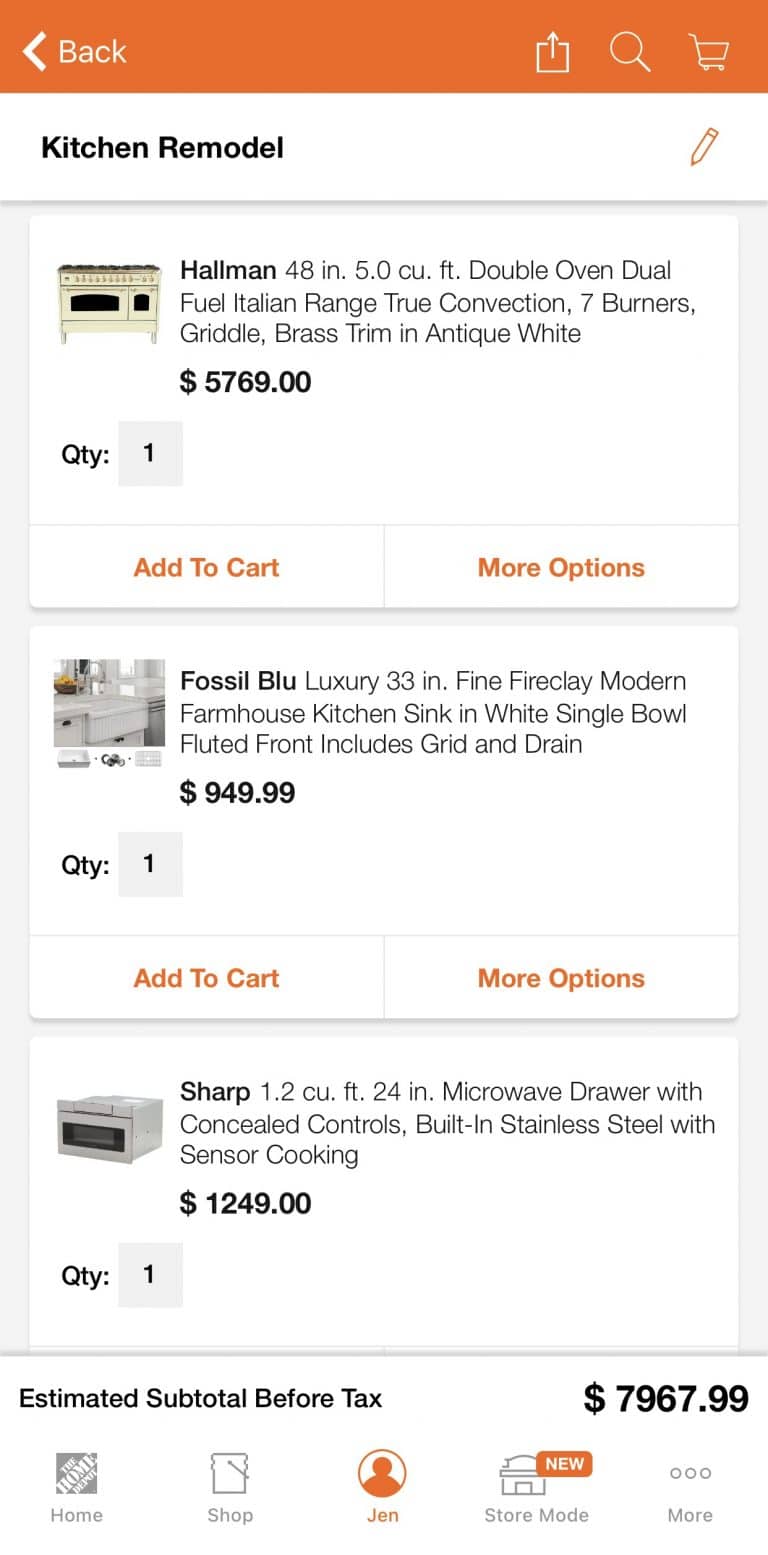This image showcases a mobile app interface related to a kitchen remodeling project. The featured section lists detailed specifications and prices of several high-end kitchen appliances and fixtures. Among the items, there is a Hallman double oven with a 48-inch by 50 cubic feet dual-fuel Italian range, including convection, 7 burners, a griddle, and antique-style legs, priced at $5,769. Another highlighted piece is a white farmhouse kitchen sink, priced at $949.99, along with a Fossil Blue luxury 33-inch reflower clay modern farmhouse kitchen sink featuring a single bowl and fluted front, although the complete description is cut off. The final item is a Sharp 1.2 cubic feet, 24-inch microwave drawer with built-in stainless steel sensor cooking and concealed controls, costing $1,249. The cumulative total for all these items is displayed at the bottom of the screen as $7,967.99.